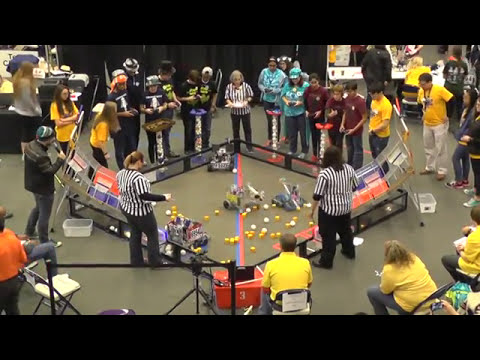The image captures an indoor scene brimming with activity, centered around a lively and competitive robot game involving remote-controlled vehicles. The focal point is a square, fenced-off stage encircled by a low, black wall and bisected by red and blue diagonal lines. Inside this arena, various robots engage in a dynamic competition involving orange and white balls. Surrounding the stage, numerous participants, many wearing bright yellow shirts, likely jury members or team members, are seated attentively. The contestants, controlling their robots from the sidelines, are also accompanied by groups donning turquoise, red, and black and yellow shirts. Overseeing the event, three referees in black and white striped shirts stand vigilantly monitoring the action. The enthusiastic crowd of about 20 people, including onlookers and participants, adds to the palpable excitement of this riveting robotic contest.